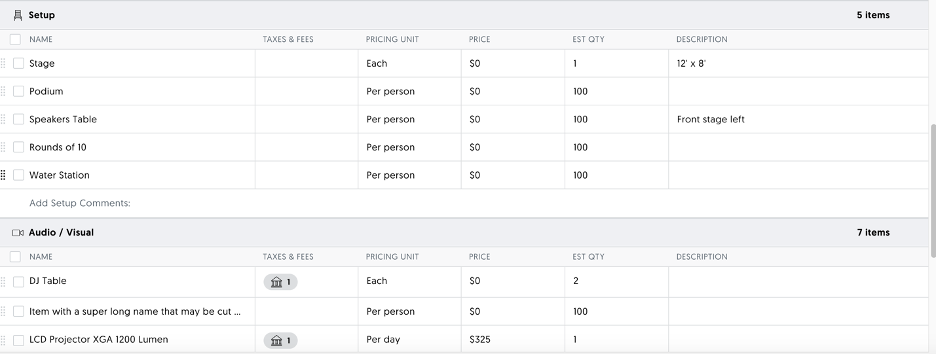The image displays a detailed event setup page featuring various sections of text and checkboxes. At the top, in black text, the title "Setup" is prominent alongside an image of a chair. The page includes several filters labeled as Name, Stage, Podium, Speakers Table, Round of 10, and Water Station. Additionally, there is a section dedicated to Taxes and Fees.

Under the Pricing Unit header, options such as "each" and "per person" are listed. The Price column shows entry fields, with the Stage's price set at $0 and an estimated quantity of 1. Other categories like Podium, Speakers Table, Round of 10, and Water Station are taxed, with each indicating an estimated quantity of 100.

Specific dimensions and positions are detailed: the Stage measures 12x8 feet and the Speakers Table is located front stage left. The second section, titled Audio Visual, features items such as a DJ Table, an item with an extended, potentially truncated name, and an LCD Projector, XDA 1200 Lumen. Notably, taxes and fees apply to both the DJ Table and LCD Projector.

The DJ Table is priced at $0 per unit with a quantity of 2, while the unidentified item is also free with an estimated quantity of 100. The LCD Projector is priced at $325 for a single unit. The page's background includes an alternating white and grey color scheme, complemented by black text.